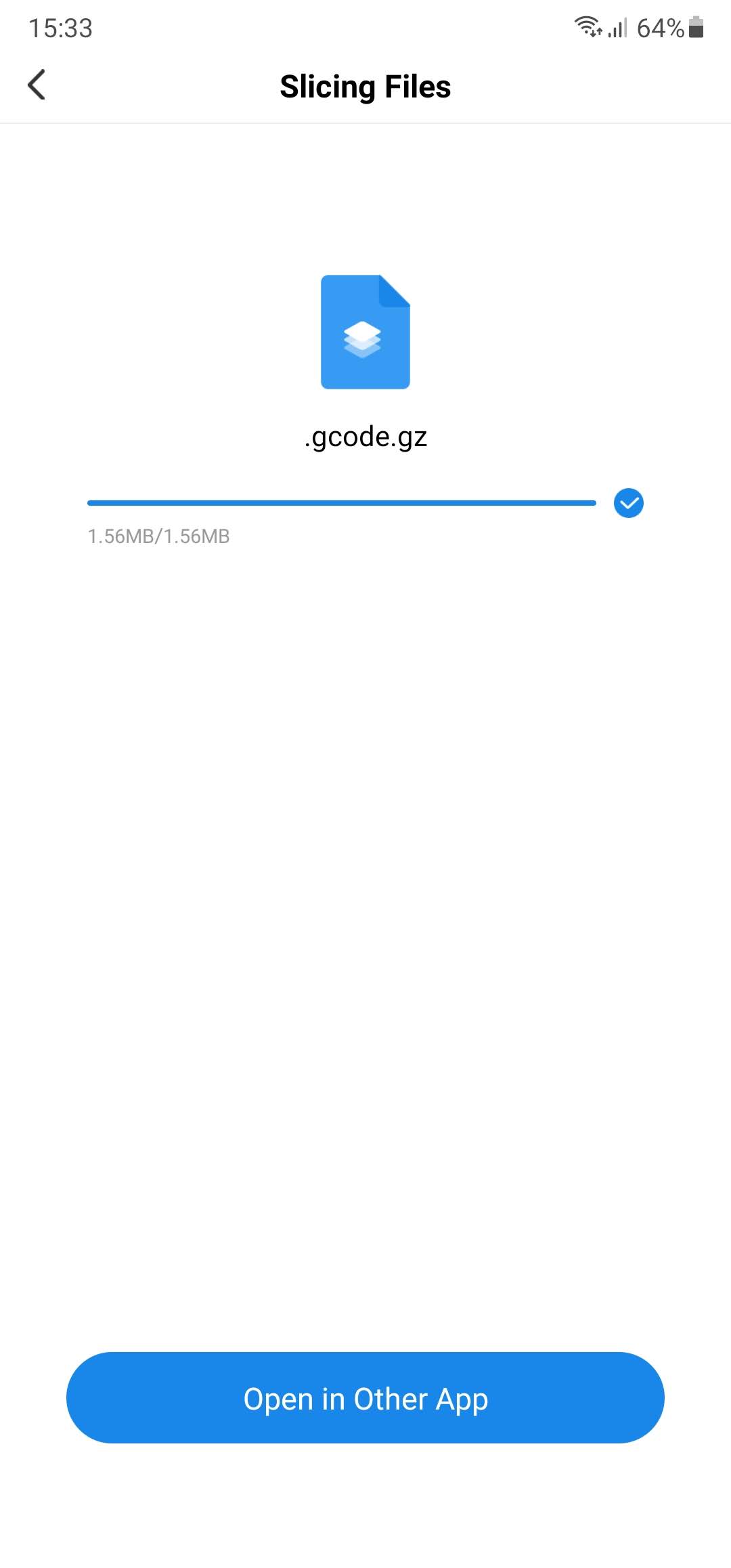The image depicts a file transfer interface with the main heading "Slicing Files" positioned at the top. An arrow pointing to the left is situated near this heading. Below it, there's an icon representing a blue page with white, stacked pages on top, featuring folded corners. Directly beneath this icon is the file name "file.gcode.gz." A status bar in blue spans across the screen, displaying a blue check mark and showing the transfer progress as "1.56 MB / 1.56 MB," indicating that the file transfer is complete. At the bottom of the screen, there is a prominent blue button labeled "Open in other app." The device's status is shown with the battery at 64% in the top right corner and the time as 15:33 in the top left corner. The overall background of the image is white and minimalistic.